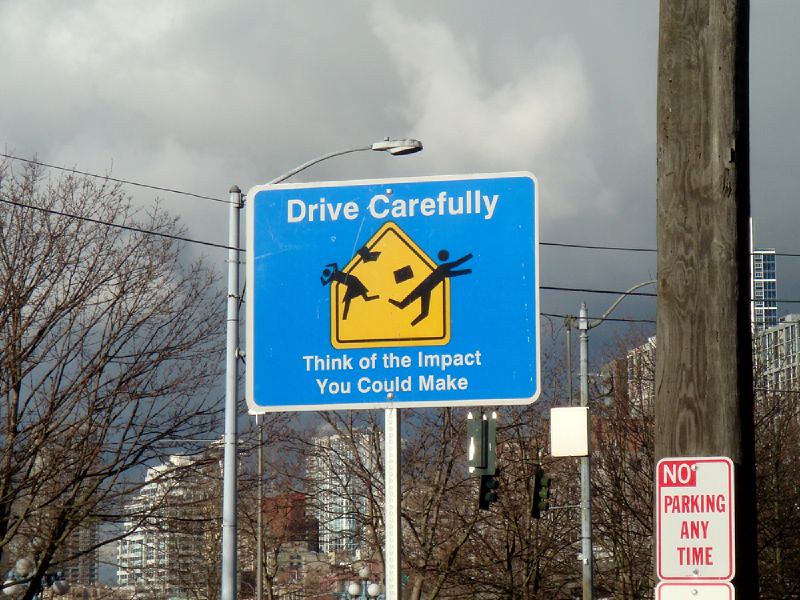The photograph showcases a bleak cityscape under a dark grey sky with lighter grey clouds. The horizon is lined with several high-rise buildings, whose view is partially obscured by tall, leafless trees, hinting at winter. Strung across the center of the image are three horizontal power lines. On the right foreground stands a thick wooden telegraph pole, or power line pole, with a rectangular white sign featuring a red border that reads "No Parking Anytime." Central to the image is a silver pole that supports a prominent street sign. The sign, mounted on a perforated steel post, features a white-bordered, blue background caution symbol resembling a schoolhouse with two pointed angles meeting at the top. The sign shows a stick figure man and woman diving out of the way, scattering books, and objects in the air, accompanied by the words "Drive Carefully" and "Think of the impact you could make," highlighting the potential danger of careless driving humorously yet poignantly. The background composition includes additional power poles, streetlights, and possibly a park area, while towering apartment buildings frame the distant skyline.